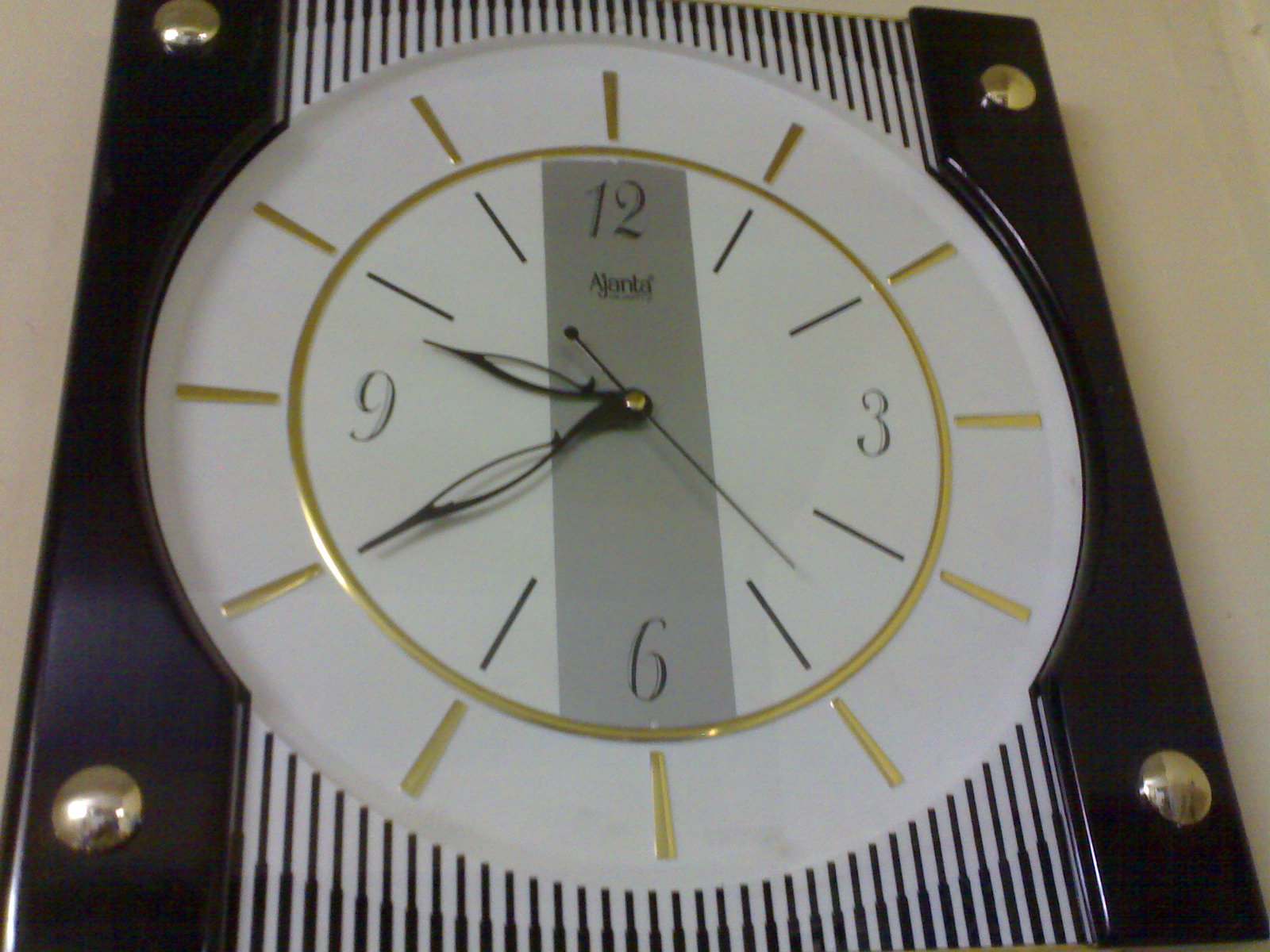This image features a detailed close-up of a sophisticated clock design. The timepiece is prominently displayed on a square mount, offering a distinctive and stylish contrast. The clock itself is round with a pristine white face, featuring elegant gold dashes and a concentric gold ring in the middle, adding a touch of luxury. Its black, pointed hands have a unique open-centered design, providing a modern twist.

The clock face includes the numerals 12, 3, 6, and 9 in gold, enhancing its readability and classic charm. A gray rectangular strip runs vertically through the center of the face, creating a subtle visual division. The brand name "Atlanta" is inscribed on the clock, signifying its authenticity and quality.

Surrounding the clock is a square mount with a black-and-white striped pattern, which appears textured and tactile. This mount is bordered by a solid black edge, each corner accented with a gold rivet, adding to the overall decorative appeal. The entire setup is mounted on a white wall, and the perspective of the photo is slightly upward and to the side, indicating the clock is positioned above eye level. The angle provides a dynamic view of the clock, emphasizing its design features and the textured mount.